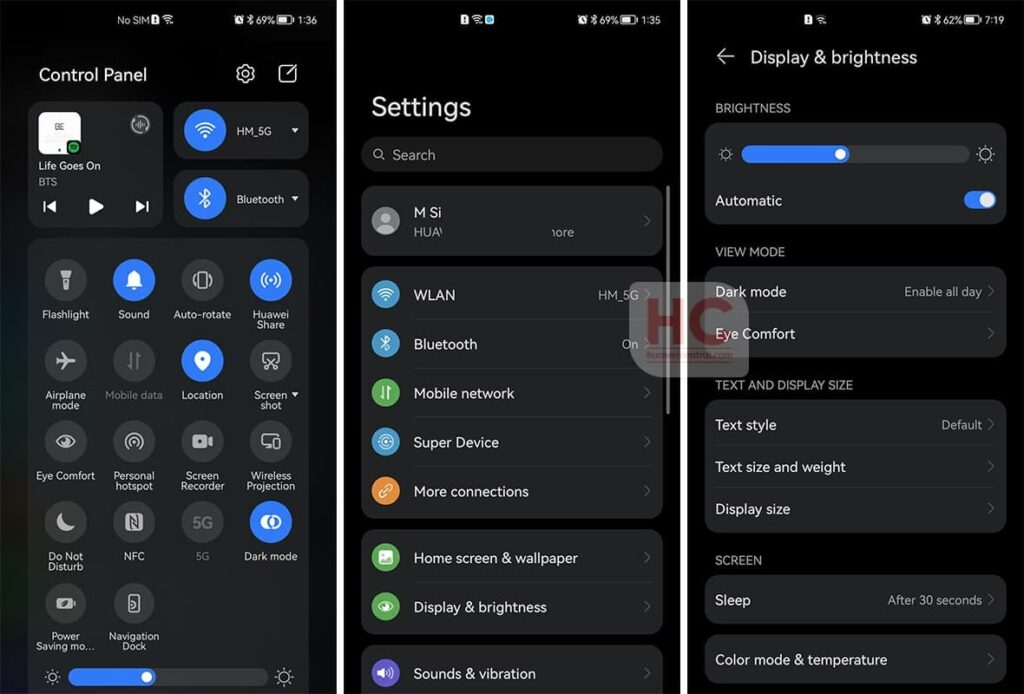This image showcases various screens of an iPhone. 

1. **Control Panel Screen**: The top of this screen displays "Control Panel" with the current time at 1:36 PM. Notifications indicate that no SIM card is inserted. Below the "Control Panel," a section reveals that the song "Life Goes On" is being played, marked by a white square icon. On the right side of the screen, an array of icons is listed from top to bottom, including symbols for HM5G and Bluetooth. Most icons are displayed in black, while those for sound, HiWoo share, and location are highlighted in blue. A long horizontal bar at the bottom of the screen provides a control for adjusting brightness.

2. **Settings Screen**: The time here is 1:35 PM, one minute earlier than on the control panel screen. A search bar labeled "MSI," though somewhat worn and not fully legible, sits below the time. A vertical list of settings options follows, featuring categories such as WLAN, Bluetooth, mobile network, super device, more connections, home screen and wallpaper, display and brightness, and sounds and vibration. Each category is marked with a round icon in various colors, including blue, green, orange, and purple.

3. **Display and Brightness Screen**: The time displayed on this screen is significantly different at 7:19 PM. The screen is titled "Display and Brightness." The brightness control is set midway, and the "Automatic" setting is turned on. Below this, there are settings for view mode, text and display size, and screen adjustments, each accompanied by corresponding control options beneath them.